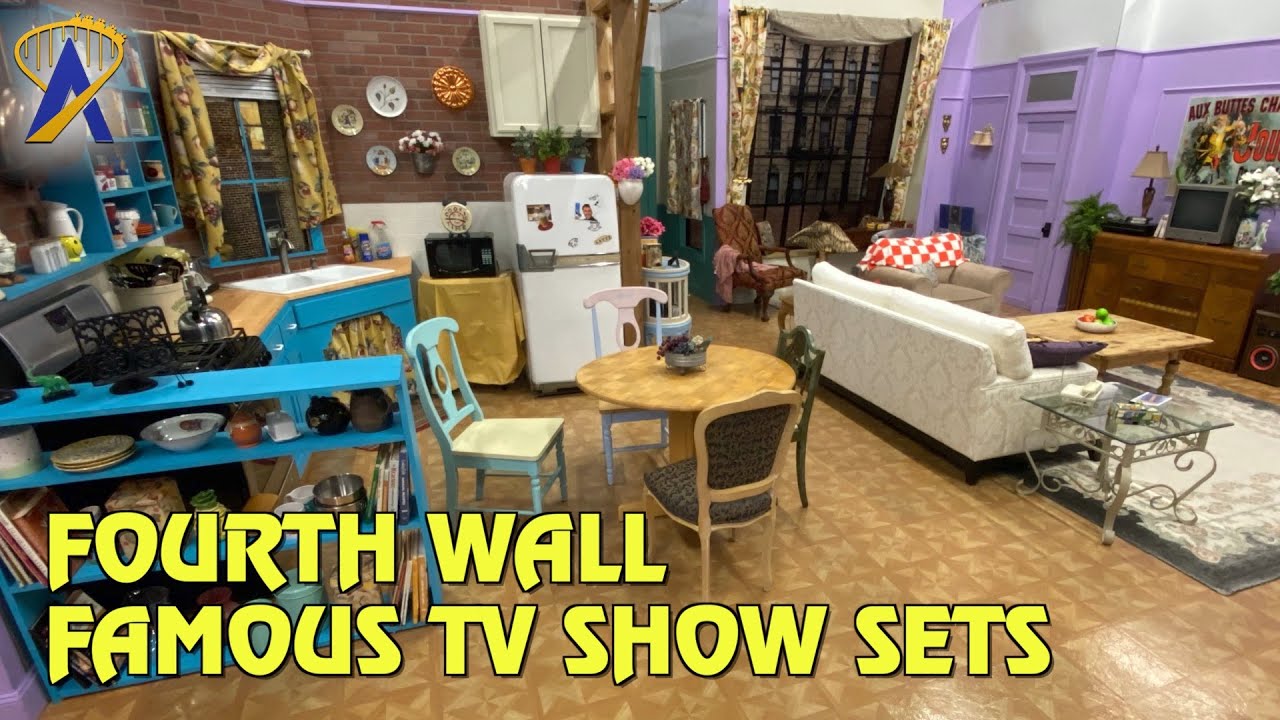This image is a realistic-looking photograph of a meticulously detailed TV show set, which could be from the famous show "Friends." The image has a horizontal rectangular shape, and in the bottom left corner, you see the caption "4th Wall Famous TV Show Sets" in big bold yellow letters outlined in black. The set resembles an apartment in the city, complete with various furnishings and vibrant colors.

The floor is a combination of light tan and beige, possibly made of tiles, wood, or vinyl. The back right wall is light purple with a band of white on top, while the back left wall is red brick. On the left side of the room, blue cabinets and shelves provide a backdrop to a kitchen area with a sink beneath a window. A white refrigerator stands in the back, topped with a small microwave on a separate small table draped with a yellow tablecloth. 

In the center of the room, a square wooden coffee table hosts some colorful food items. Near the coffee table is a white couch facing a small grey television sitting on a brown cabinet that also holds a lamp. In front of the cabinet lies a white rug on the brown floor. Behind the couch stands a circular dining table with mismatched chairs around it. A brown armchair with a white and orange checkered blanket is also visible. Dishes, utensils, and kitchen appliances, such as a stove with a kettle, further emphasize the domestic setting. The bottom left foreground of the image features a turquoise bookshelf, adding more character to the room. Overall, the set is intricately designed to resemble a lived-in apartment, rich in detail and quintessential of iconic TV show environments.